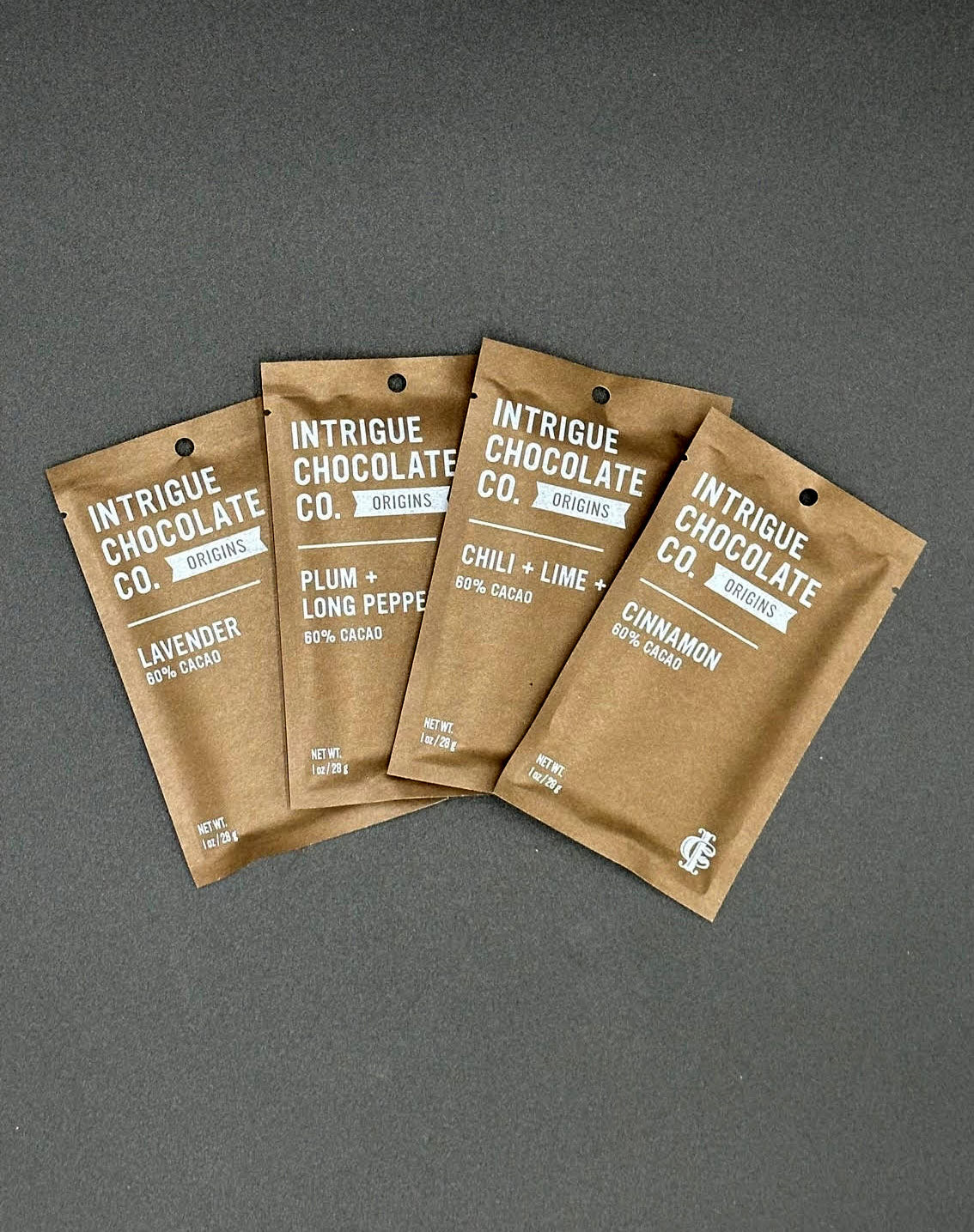The image features a gray background with four brown packages of chocolate from Intrigue Chocolate Company, each placed side by side. The packages are labeled in white letters with different flavors: lavender, plum & long pepper, chili & lime, and cinnamon. Each packet has a net weight of 1 ounce (28 grams) and displays the company's name, Intrigue Chocolate Co., at the top in white text. An emblem with the letters "I" and "C" encased in a circle appears on the lower right-hand corner of each packet. The chocolate packets also indicate a cocoa content, with the cinnamon, chili & lime, and lavender varieties listed as 69%, while the plum & long pepper variety is listed as 60%. The packets are neatly arranged and the flavor labels are prominently featured.